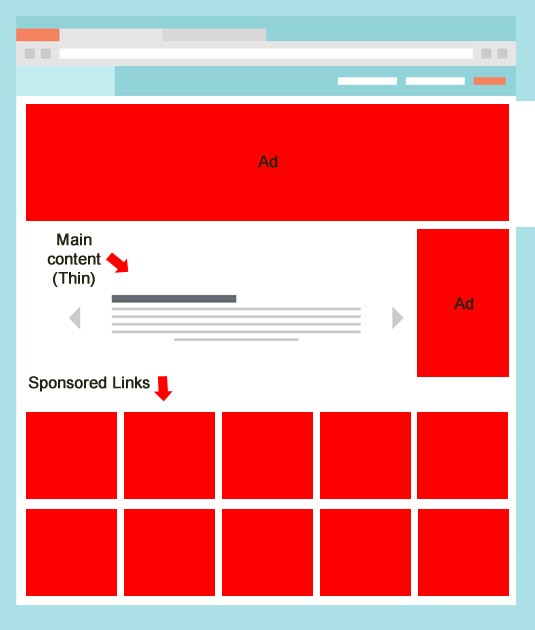The image captures a screenshot of a webpage layout, emphasizing its potential for advertisements. The browser window, outlined in light blue, features a silver search bar at the top. The main content area is dominated by various red rectangles and squares, indicating spaces reserved for ads rather than actual advertisements. 

At the upper section of the page, instead of a typical header, there's a red rectangle labeled "ad" in black text. The right sidebar, also comprised of ten smaller red squares, similarly labeled "ad," further underscores the ad-heavy design of this layout. Positioned at the bottom of the page, a white background with black text reading "sponsored links" points downward toward the ads above.

Centrally located on the page is a white rectangle with a label indicating "main content," accompanied by an arrow pointing towards it. Beneath this label, "thin" is written in parentheses, highlighting that a minimal portion of the webpage is allocated to actual content amidst the overwhelming ad spaces.